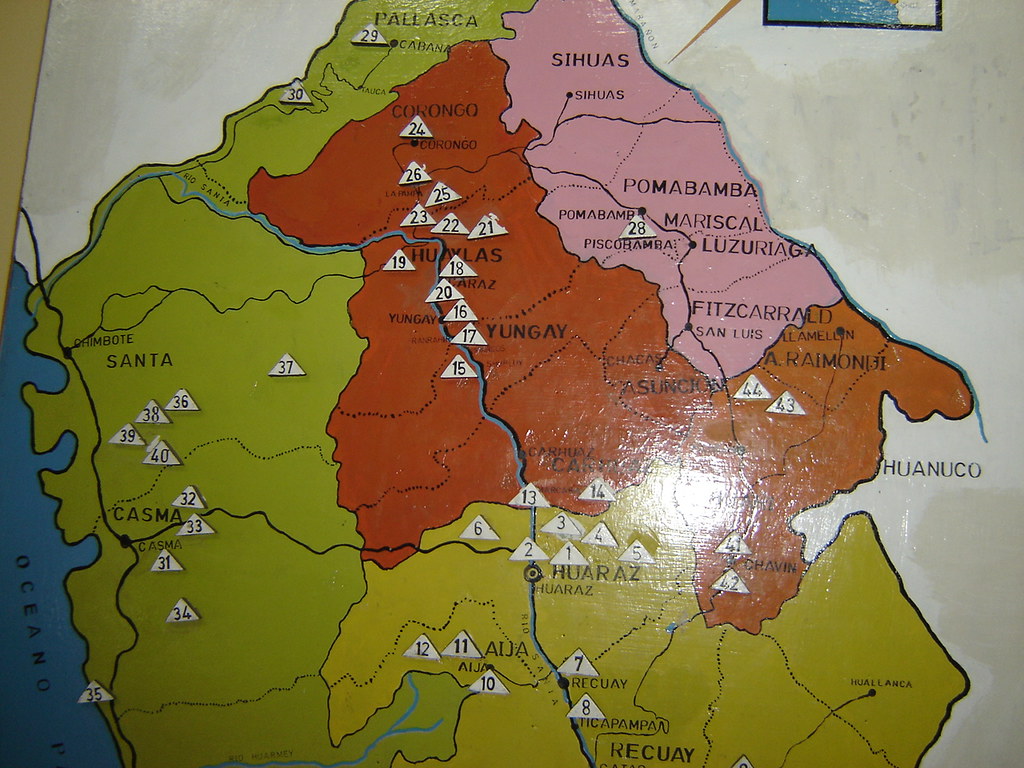This photograph depicts a detailed, full-color map displayed on a white background. The map, possibly on a wall for display, features a diverse palette with each area demarcated distinctly: green for Santa and Casma to the left, brown for Yungay, and an army green-yellowish hue for Huarez. The map is carefully segmented: a pink section at the top right names Poma Bamba, and in the green sections are both Santa and Casma. A prominent blue line, likely a river, runs vertically through the center, paralleled by numerous white triangles with numbers inside. The map also shows a flash spot at the center from a camera, which briefly obscures part of the image. To the left, the area is labeled Ocean, emphasizing its coastal aspect. The different colors and meticulously printed names, including places like Juanuco, Huatz, and other regions, enhance the readability and visual appeal of the map.